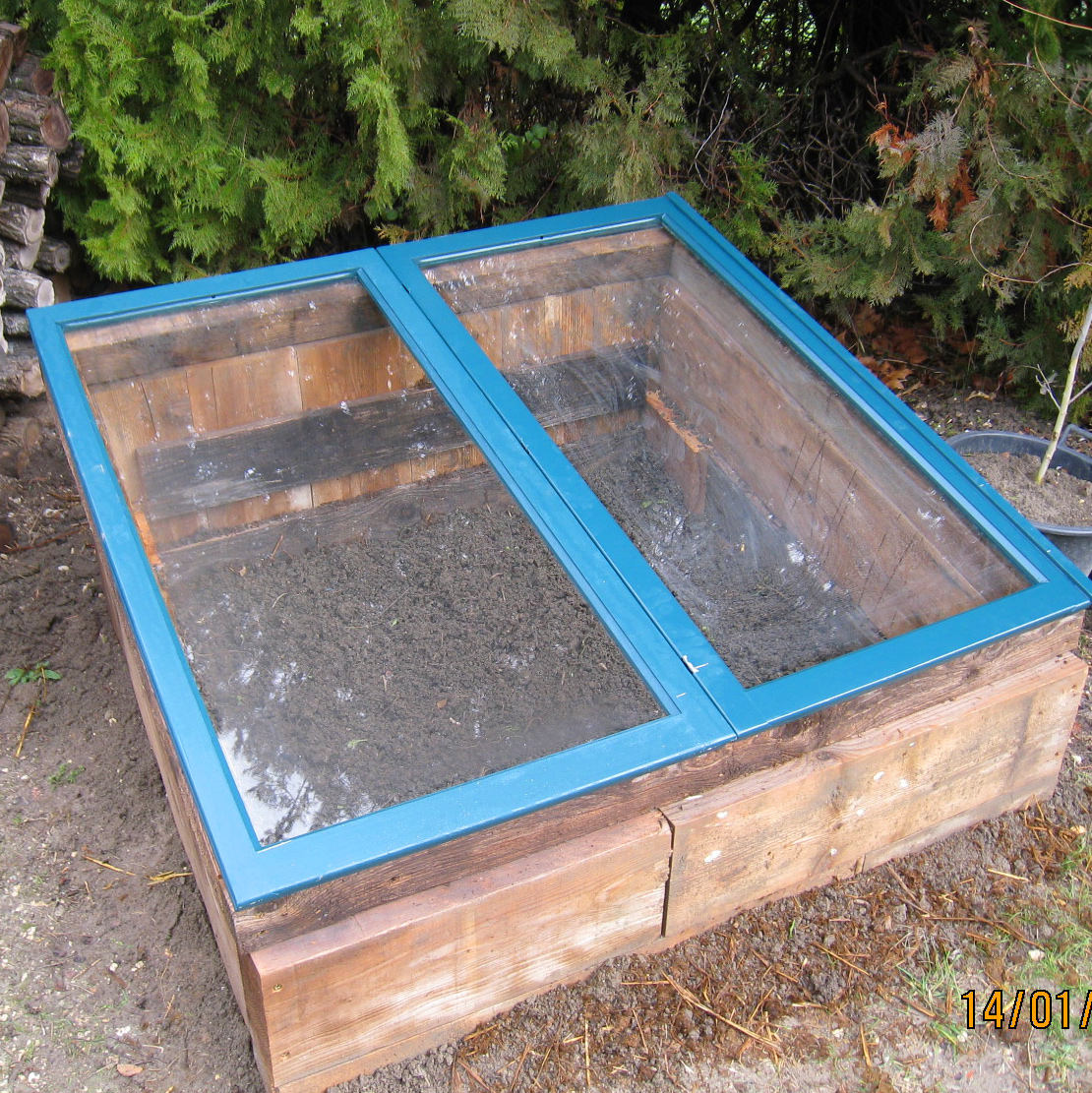In this image, we see a uniquely constructed wooden and glass box situated on top of dirt, all set against a backdrop of coniferous, needly shrubs. The box is made from weathered, possibly one-by-eight planks nailed or screwed together to form a square base, which is open at the top. The open top is framed by blue-painted wooden rectangles inset with glass panes, resembling a cabinet lying on its side with an exposed bottom directly interacting with the soil. 

The wooden box, tilted slightly to the left in the picture, features supporting planks at the top and bottom, suggesting a sturdy frame. To the left background of the image, there is a small stack of grayish wood, while to the right, another similar plant is visible next to a pot containing a small tree. This garden setting implies utility, and the box might serve as a vermiculture bin, designed to facilitate the decomposition of plant scraps by worms to produce compost. However, it lacks the typical air vents found in larger composting systems indicating a more compact and potentially specialized purpose. The ground beneath is grayish with organic material, and the photo is timestamped "14/01" in the lower right corner.